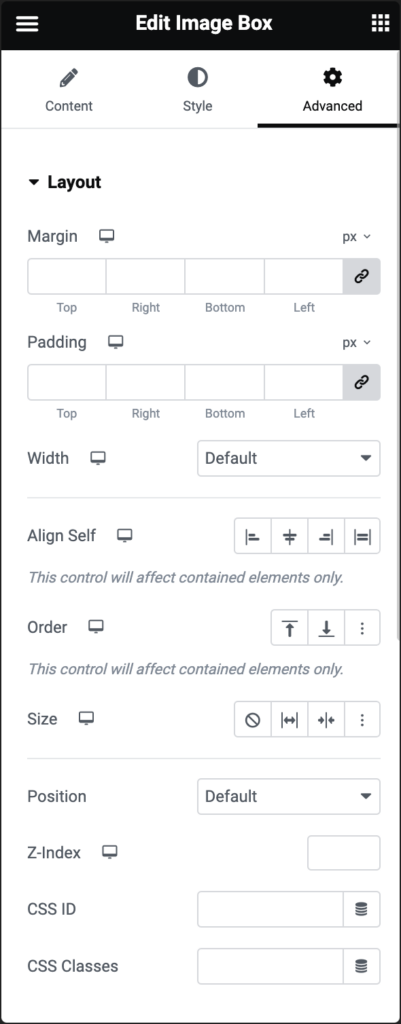In this detailed image, we see an editing interface. At the top is the title of the section. Beneath the title, there are three neatly arranged tabs: "Content," "Style," and "Advanced." The "Content" tab is marked with a pencil icon, indicating its function related to textual or media content editing. The "Style" tab is represented by a half white, half dark gray circle, signifying design or visual appearance customization. The "Advanced" tab features a gear icon, likely for more technical or in-depth settings.

Directly below these tabs is a section dedicated to layout settings. The first option is for adjusting the margin, with input fields for the top, right, bottom, and left margins. Following margin adjustments, there are controls for padding, which similarly allow inputs for the top, right, bottom, and left padding settings.

Subsequently, the width setting is displayed, with the option currently set to "default" on the right side. Continuing below, there is an "Align Self" control that includes a note specifying that this control will only affect contained elements, ensuring alignment adjustments are applied solely to nested components. Finally, there is an "Order" option, which also features the same note, indicating it influences the sequence of contained elements only.